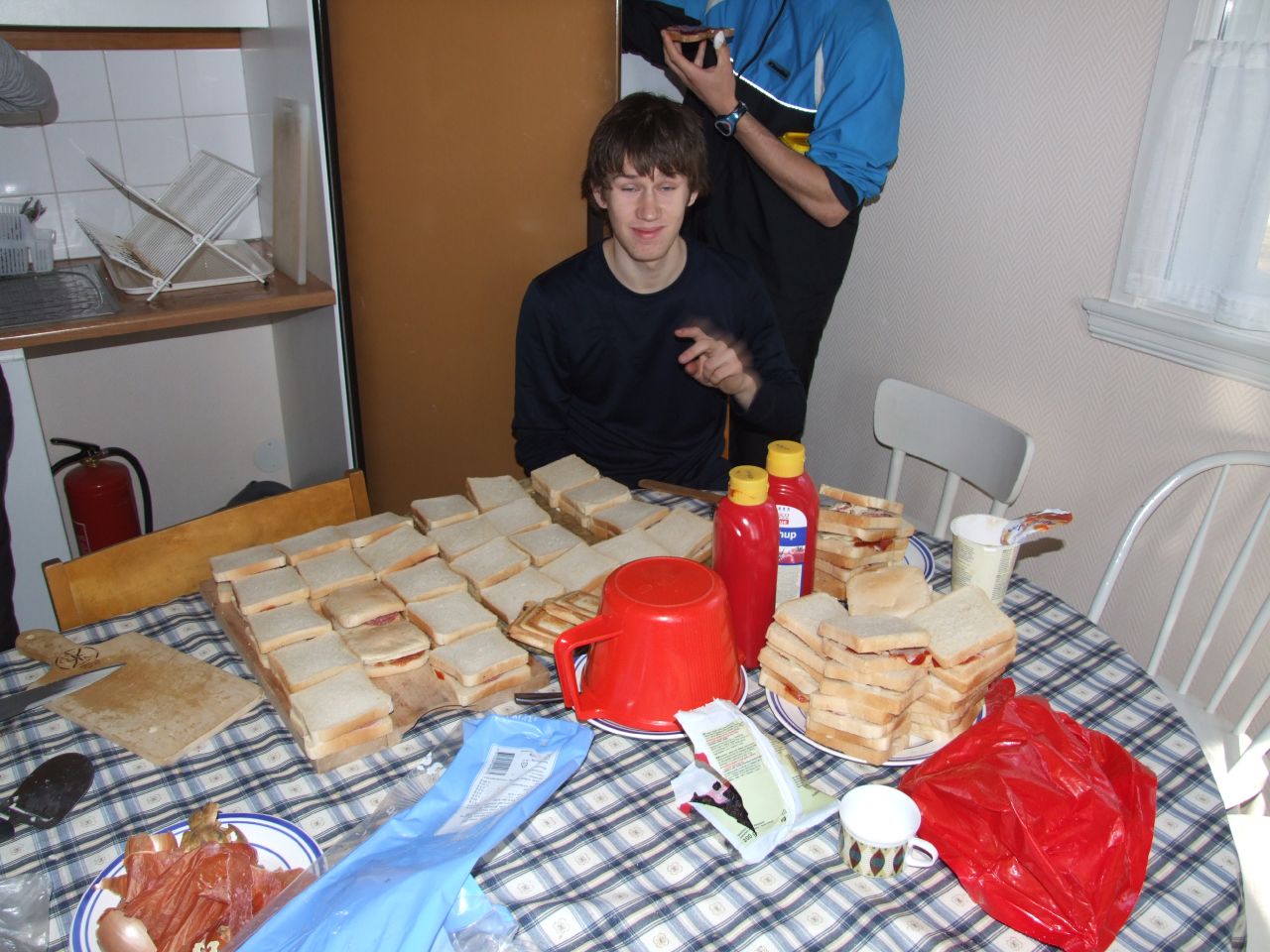In the image, a white man with brown, longer hair sits at a kitchen table covered with a blue and white checkerboard tablecloth. He is busy making sandwiches, which are meticulously lined up on a large cutting board and a round platter, with some sandwiches stacked on one side. The man, dressed in a blue shirt that transitions from light blue at the top to darker blue at the bottom, holds a piece of bread in his left hand above the table, while his right hand is not visible, positioned below the table. Beside him, another person stands, partially out of frame, with only their body visible.

Around the table, which is surrounded by mismatched chairs, are various items: a plate of raw bacon, a black wallet or similar object, an empty cutting board, a red bag, a cup, a water glass, and a paper cup with something in it. Two bottles of red sauce, likely ketchup, with yellow tops, and an upside-down red bowl with a handle are also on the table. The kitchen background features a dish drying rack, a fire extinguisher, and a window. The walls are tan on one side and adorned with white tiles on the other.